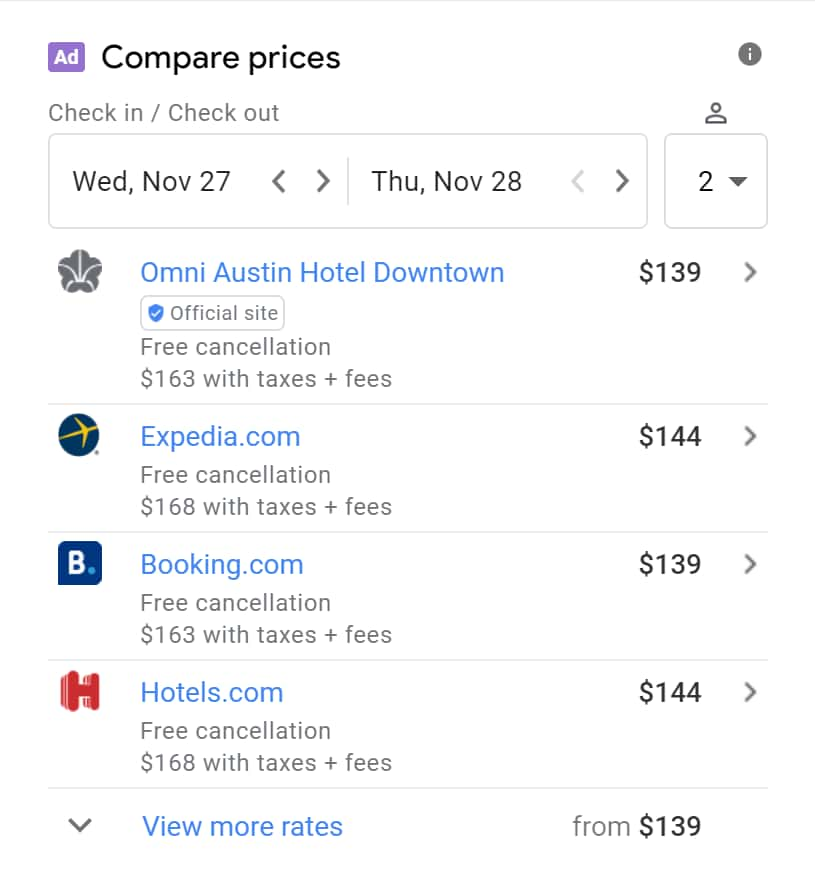The image displays a section of a travel comparison website, specifically highlighting its advertising feature. At the top, the website prominently states "Compare Prices," inviting users to evaluate various travel costs. The user interface includes a search bar where visitors can input their travel dates and the number of travelers to tailor their search.

Displayed prominently are several booking options for the Omni Austin Hotel Downtown from well-known travel websites, including Expedia.com, Booking.com, and Hotels.com. Each booking option shows the total price, inclusive of taxes and fees. Additionally, there's an option to view more rates from other companies. 

A consistent message below each price reassures users with the offer of free cancellation if they book through any of the listed providers. This feature aims to provide users with a comprehensive and convenient way to find the best travel deals, ensuring both cost transparency and flexibility in booking.